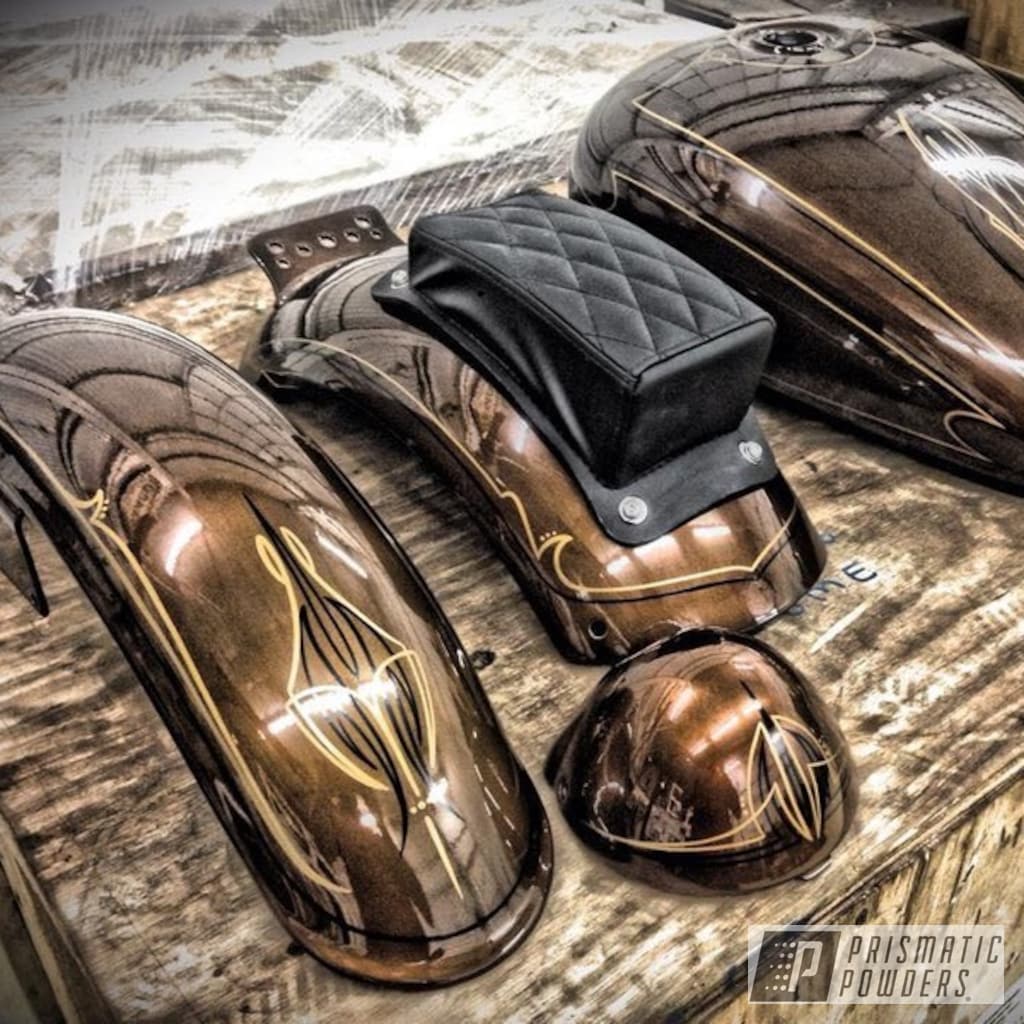The photograph, taken indoors, showcases various components of a motorcycle laid out on a large plywood crate. Central to the image are disassembled parts, including a fuel tank, front and rear fenders, a headlight cover, and a cushioned rear fender. Each piece features a striking metallic bronze-gold base coat adorned with intricate black, white, and yellow lines. To the left, a fender curves gracefully, its shiny finish catching the light. Adjacent to it sits what appears to be a headlight cover. To the right, the fuel tank and a piece with a black leather cushion, presumably the rear fender, are prominently displayed. At the bottom right corner of the image, a semi-transparent logo reads "Prismatic Powders," marked by a distinctive emblem that looks like a pea against a black background with white dots emanating from it. The detailed craftsmanship and cohesive color scheme suggest a high-quality custom painting service for motorcycle parts.